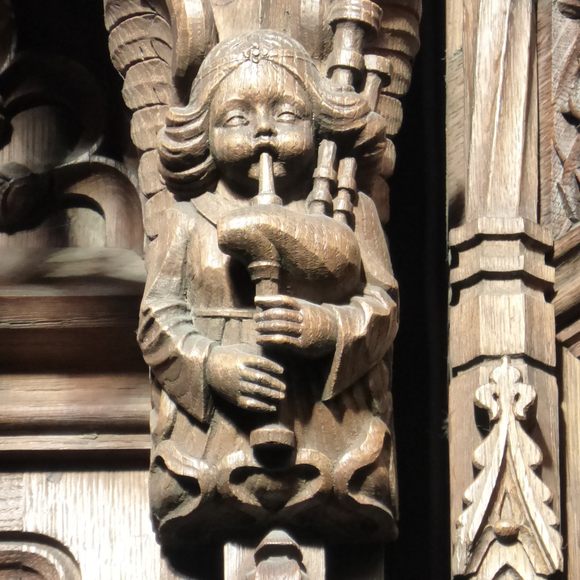This square, color photograph captures a highly detailed wooden carving, likely part of an ornate structure such as a chapel or valuable piece of furniture, possibly a china cabinet or dresser. The carving features a young girl with flowing hair that spills out from beneath a hat, dressed in a garment adorned with heart-shaped carvings at the hem. She is depicted playing a set of bagpipes, with her cheeks puffed out and lips pursed in mid-blow, while her hands are positioned on the lower part of the instrument. The wood has a rich, copperish golden hue, enhanced by the natural light that bathes the scene, suggesting it could be taken either outdoors or indoors with ample lighting. Behind her, the stained wood background further accentuates the intricate details of the carving, which includes additional ornate imagery, such as patterns resembling Christmas trees. The setting evokes a sense of sacred or significant artistry, reminiscent of what one might find in a church or cathedral.